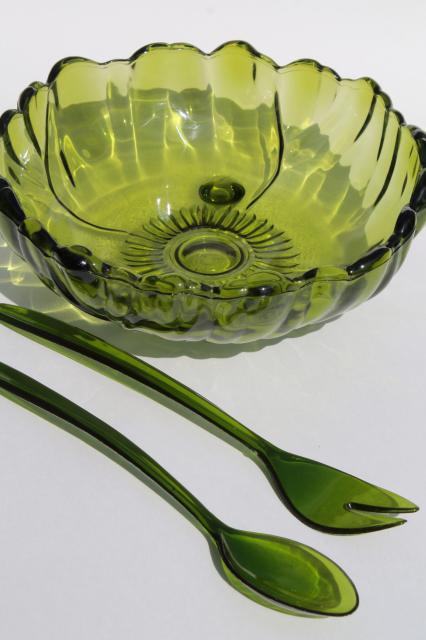The image features a vintage-looking, translucent avocado green glass bowl and a matching salad utensil set, comprising a long-handled spoon and a distinctive fork with two close-set prongs. The bowl displays a unique design with scalloped edges, resembling a flower or a cabbage leaf with wavy contours, and includes a sunburst pattern in a darker shade of green at its center. The utensils, designed for serving salad, share the same green glass material. The background of the image is plain white.